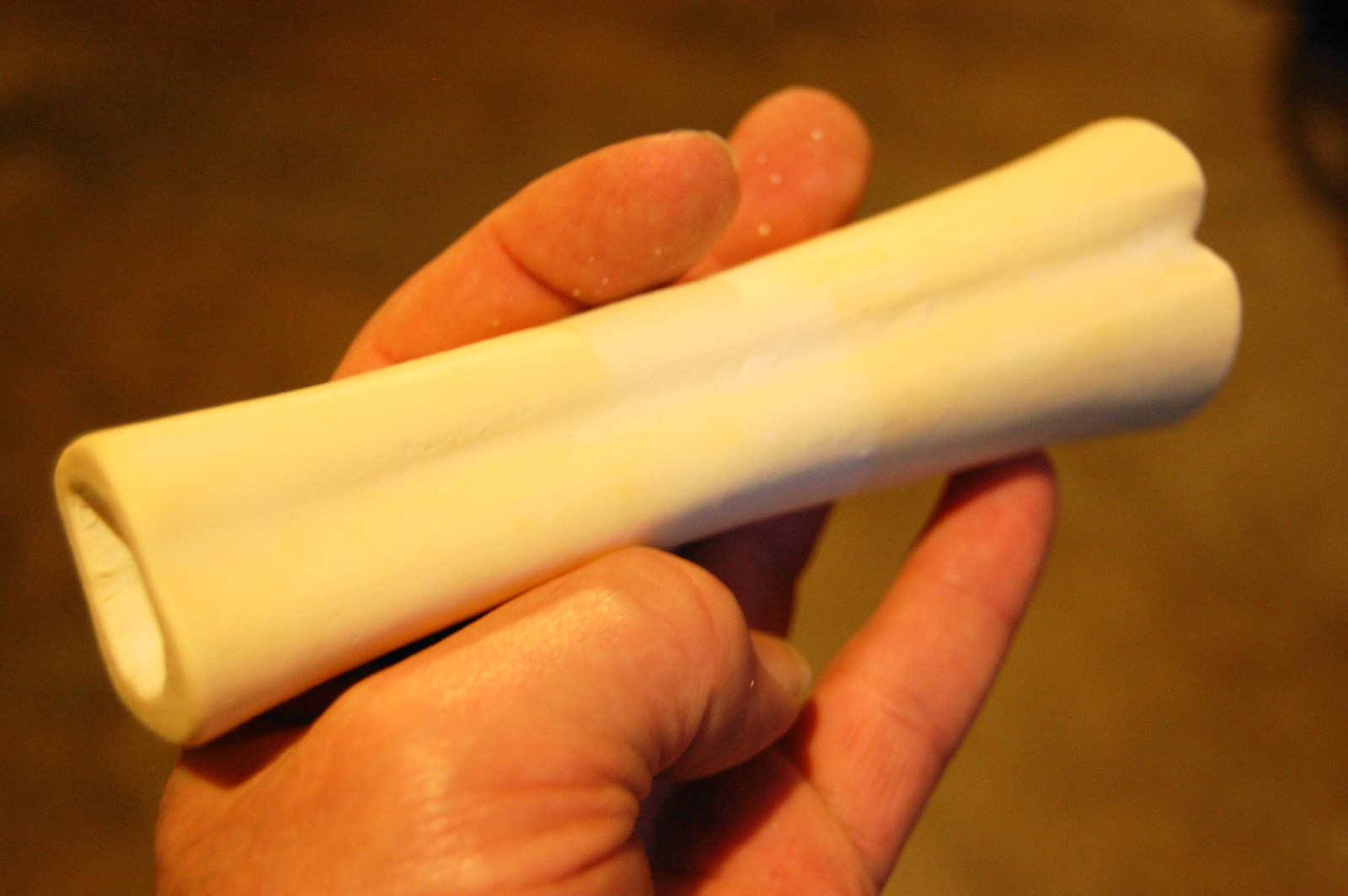This is a close-up photograph of a man's left hand holding a smooth, hollow dog bone snack in an awkward position. The bone, about eight inches long, is a bleached-out white color and has flakes on the man's fingertips, suggesting it might have been polished or sanded. The man's thumb is curled under the bone, with the thumb tip tucked in, while the pinky and ring finger support the bone from underneath. The pointer finger is slightly wrapped around it but curved inwards, and the middle finger is slightly extended away. The background is a blurred tan color, possibly dirt ground, with a round and black object, likely a piece of machinery, visible in the upper right. The overall lighting of the image has a yellow cast, highlighting the cream edges of the bone and the Caucasian skin tone of the hand.